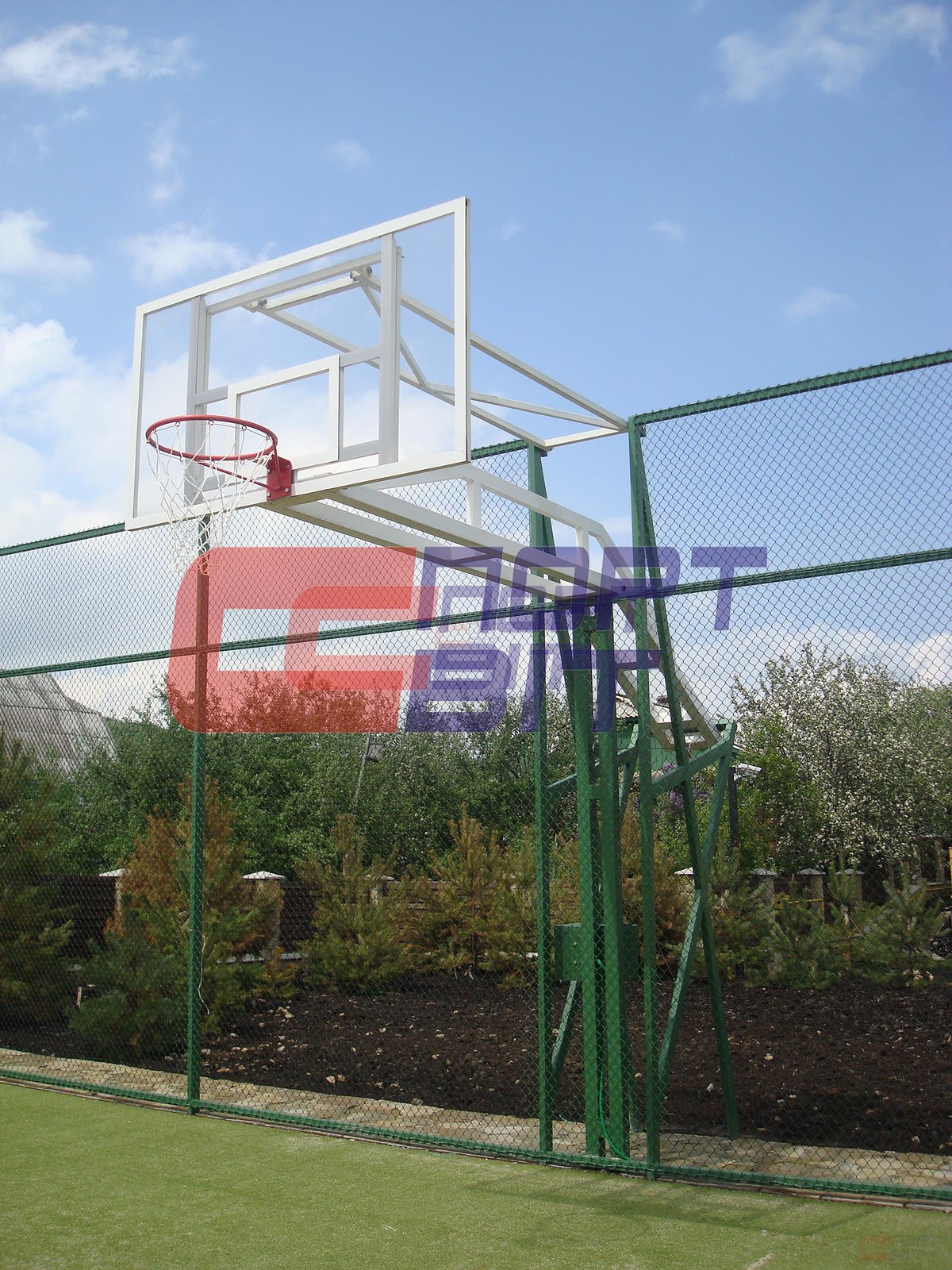The image depicts an outdoor basketball court with a clear backboard framed in white and an orange hoop and net attached. The court itself is covered in green AstroTurf, surrounded by a tall, deep green chain-link fence with green metal posts, likely designed to prevent basketballs from escaping the area. Though there is a slightly blurry text overlay in the center of the image, reading something like "C-...-O-P-T ... B-I-T," it doesn't provide any clear information. The background reveals a beautifully landscaped park with a mulch-covered ground, bushes, and a path adorned with posts and lights. To the left, a structure that appears to be the top of either a greenhouse or a solar array is visible. The day is clear with a blue sky and puffy white clouds, suggesting it’s sunny and bright.